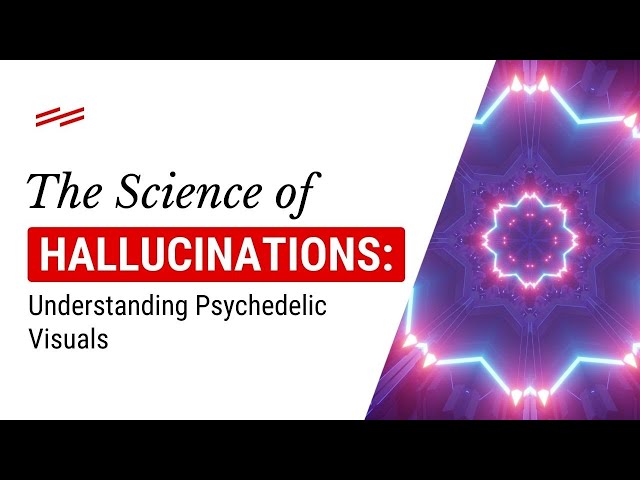The image features a visually striking composition focused on the theme "The Science of Hallucinations: Understanding Psychedelic Visuals." On the right-hand side, there are intricate geometric shapes resembling octagons, dynamically interlocked with one another. These shapes are rendered in an array of colors including dark and light purple, light pink, light blue, red, black, and white. To the left, the text is prominently displayed, with "The Science of Hallucinations" in black text, while "Hallucinations" stands out in white text against a red background, and is followed by the subtitle "Understanding Psychedelic Visuals." The entire scene is framed with black borders on the top and bottom, giving it a polished, banner-like appearance. Lines of varying thickness and colors are scattered, particularly in the top left corner, enhancing the image's complexity. The overall style suggests it could be the cover slide for a presentation designed to educate viewers on the nature of psychedelic hallucinations, using a blend of scientific and science fiction-inspired visuals.